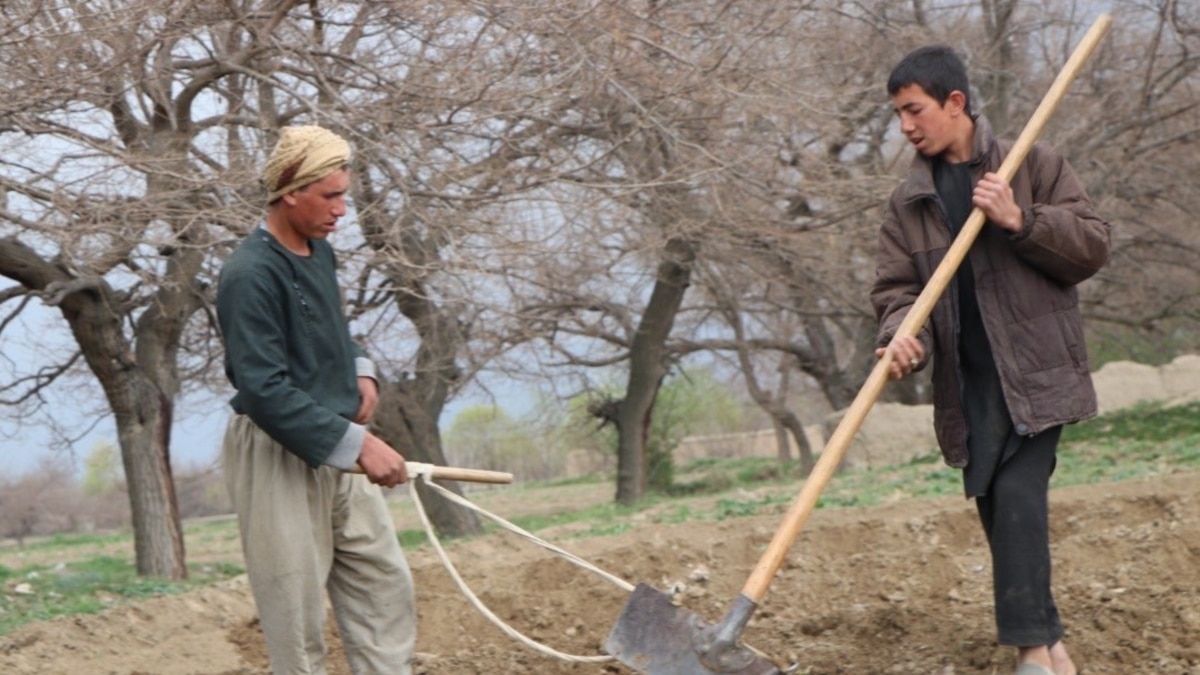The photograph captures a poignant scene of two individuals, seemingly a father and his teenage son, working diligently in an outdoor, barren field. The older man, with a tan bandana tied around his head, wears a long-sleeve green shirt paired with tan cloth pants and appears to be using a hand tool to tend to the soil. The younger boy, approximately 16 years old, sports a brown puffer jacket over a black shirt with black cloth pants and grips a large, shovel-like tool for digging. Both individuals have medium skin tones and somber expressions, reflecting the arduous nature of their task. The soil they are working on appears infertile, and no crops are visible, suggesting that they are preparing the ground for future planting. The surrounding landscape is stark, with a line of tall, leafless trees marking the colder season. The sky above is cloudy, further heightening the photograph's melancholic atmosphere. The image quality is somewhat grainy, lending it an almost vintage feel, though it may be a contemporary capture of a challenging moment in their agricultural endeavors.